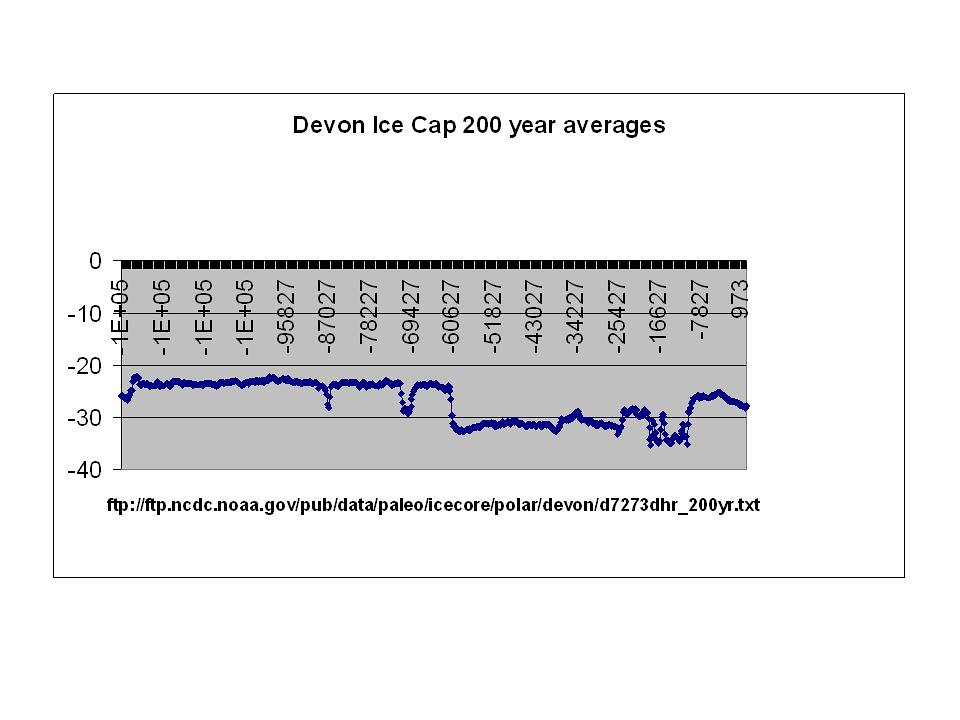The image features a detailed graph titled "Devon Ice Cap 200-Year Averages," set against a white background. The graph's primary structure is a gray bar running vertically, with a blue line graph plotted within it. Along the left side of the graph, black numerical labels indicate temperature values at intervals of 0, -10, -20, -30, and -40 degrees. The graph depicts numerical sequences along the horizontal axis that include scientific notation and numeric values, such as 1e+05, 1e+06, -95827, and -87027, among several others. The blue line graph is composed of diamond-shaped data points, illustrating temperature trends over the specified period. The bottom of the graph includes a link to the National Oceanic and Atmospheric Administration's (NOAA) website, although the link itself is quite lengthy.